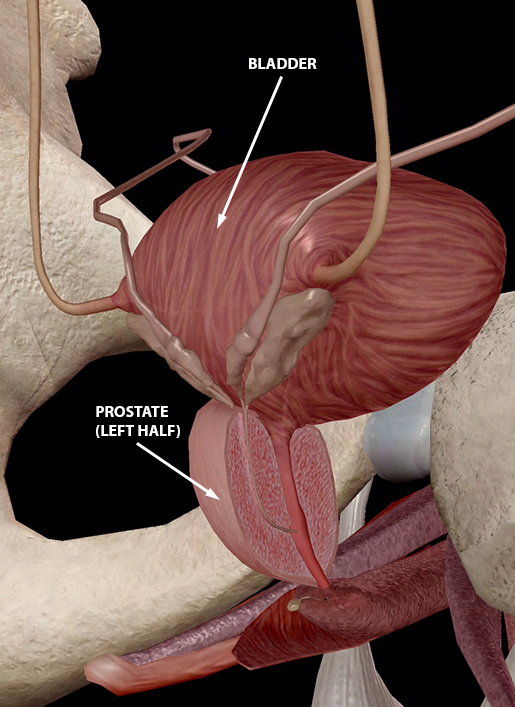This detailed close-up diagram of a human bladder, taken from a medical text, provides a comprehensive view of the urinary system with emphasis on the bladder and prostate. The central feature is the bladder, identified by white text on a black background with an arrow pointing to a red, fleshy organ marked by pink lines. Surrounding the bladder are intricate tubes or vessels, likely blood vessels, that extend from it. Beneath the bladder, the diagram highlights the prostate, labeled in white text as "prostate (left half)," with an arrow indicating its location. The prostate appears as a large, light pink, fleshy area. The diagram also includes beige and white bones with shadows, likely representing the pelvic bone, with noticeable holes and black shading. The muscles are predominantly red with pink splotches, and tendons connecting upward from the bladder are rendered in pink or beige. The overall color scheme is predominantly black, red, tan, light pink, and dark red.